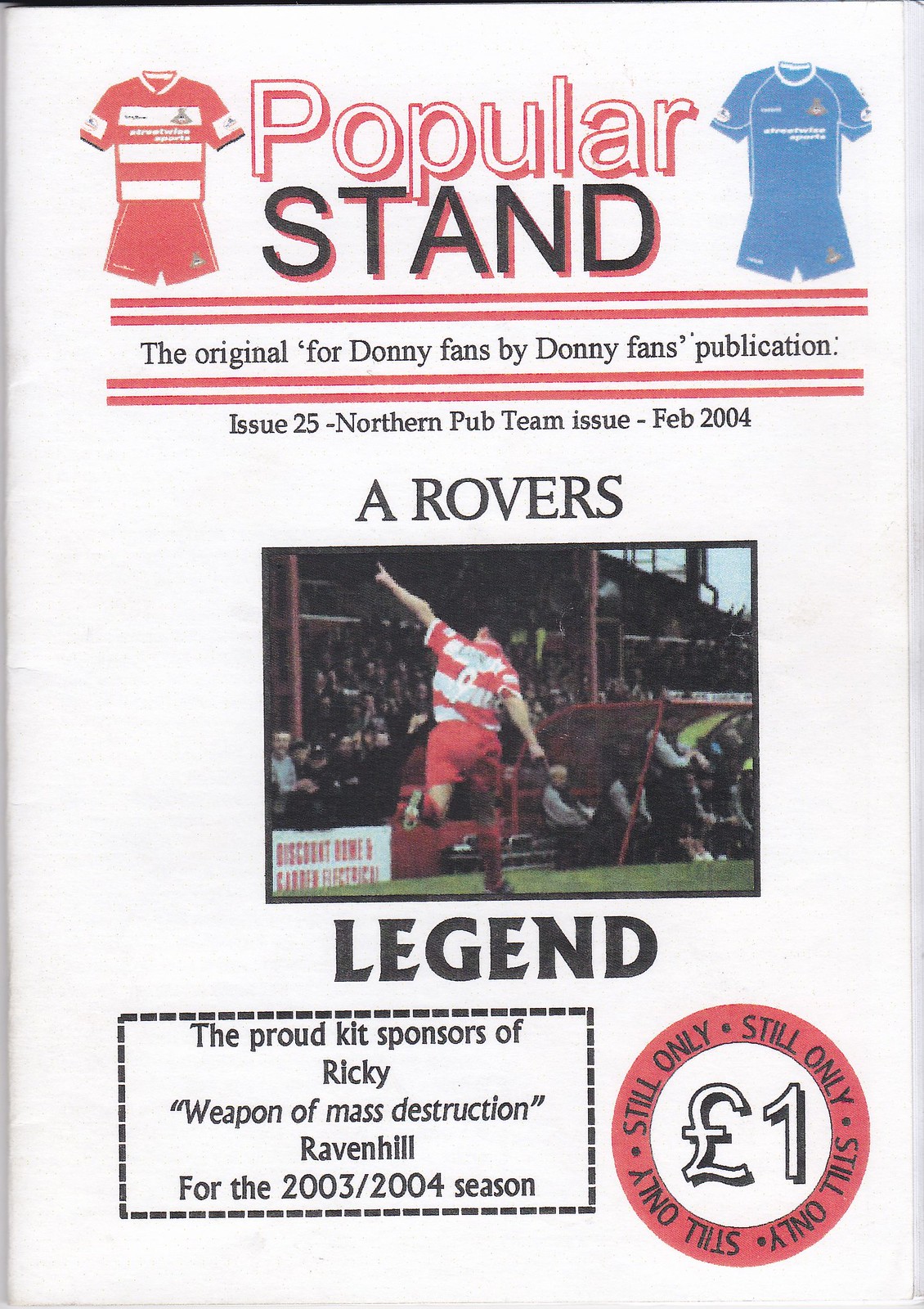The front page of the program or magazine features a clean white background, with "Popular Stand" prominently displayed at the top. Flanking the title are two soccer uniforms: to the left, a red and white kit, and to the right, a blue and white kit. Below this title, two horizontal red lines with a white line sandwiched between them frame the text: "the original for Donny fans by Donny fans publication."

Further down, another similar horizontal line border encloses the text: "Issue 25, Northern Pub Team Issue, February 2004." Immediately below, the words "A Rovers Legend" are centered, with "A Rovers" and "Legend" appearing above and below a dynamic image of a soccer player dressed in red shorts and a red and white striped jersey. The player is depicted with an arm raised, seemingly in motion on the field. The bottom of the page notes, "Proud kit sponsors of Ricky 'Weapon of Mass Destruction' Ravenhill for the 2003-2004 season."